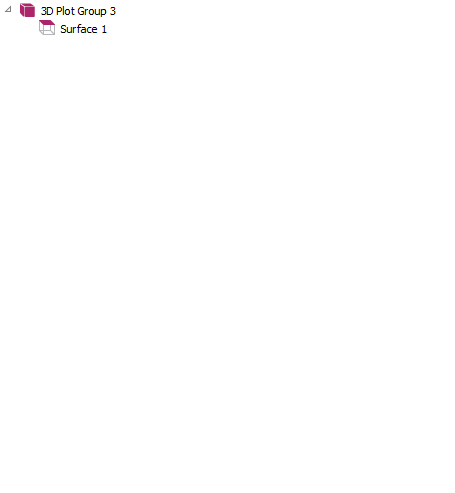The image appears to be a screenshot from a 3D modeling or graphical program, possibly Blender, 3D Studio Max, or Modo. The image is predominantly a blank white canvas, occupying the majority of the space. 

In the upper left corner, there is a minimalistic diagram consisting of a white, borderless background. Here, a triangle is depicted with a flat base along the bottom, a vertical line on the right, and a hypotenuse stretching from the lower-left to upper-right. 

Adjacent to this triangle is an isometrically-drawn cube. The cube is purple with gray outlines, suggesting a wireframe model. 

Directly next to this cube, there is text that reads "3D plot group 3." Below this text is another inset of the same cube, but in this instance, only the top surface remains purple while the rest of the cube is represented by gray lines, showing the front, bottom, and back faces. This smaller cube is labeled "surface 1," indicating it as a subset or specific section of the previous cube.

The remainder of the image is a plain white background, which could easily be covered with a thumb, highlighting the minimalist design and focusing attention on the small diagrams and text.